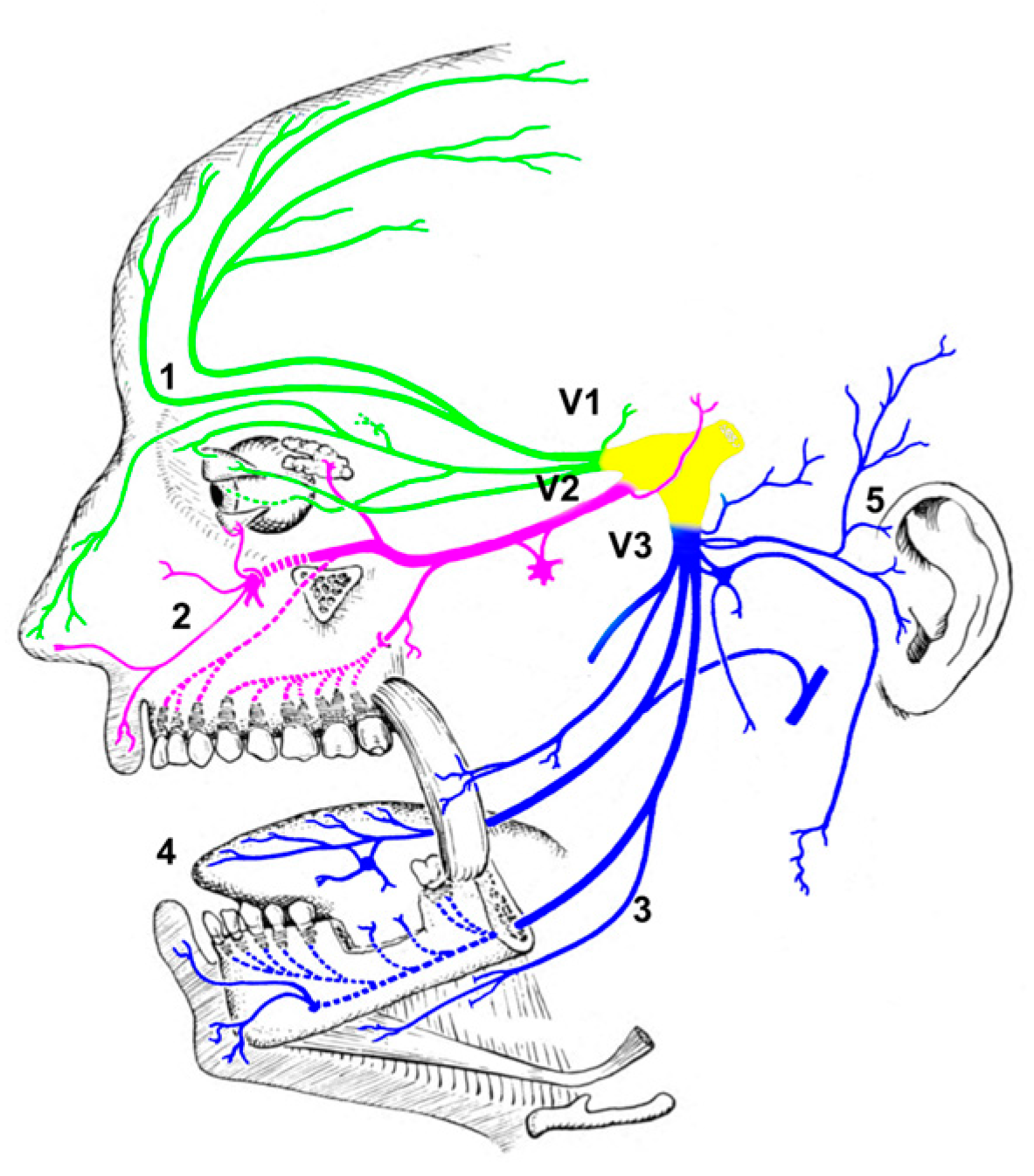This detailed medical illustration depicts a human head in profile, facing left, outlined in black and white against a white background. The ear, situated on the right side of the image, is detailed in black and white. Various networks of color-coded vessels or nerves are prominently displayed throughout the head and are labeled V1, V2, and V3.

The V1 network is illustrated in green. This network originates near the temple and extends toward the forehead, then curving back to the top of the head like streets. It further extends to the tip of the nose, the upper eyelid, and the eyeball.

The V2 network appears in fuchsia or pink and extends from a central hub near the temple. It feeds into the upper teeth, possibly the sinus cavity, the upper lip, and the nostrils. It also travels beneath the eye to some kind of gland or structure behind the eye.

The V3 network, depicted in royal blue, stretches from the temple to the ear, continuing above and behind the ear, and down towards the chin and tongue. It displays connections to the ear, lower jawbone, lower lip, lower teeth, and the tongue.

Central to these networks is a thick, yellow T-shaped area at the temple, which acts as a hub from which all the colored lines originate. The eye in the illustration is shown in black and white, as are the teeth, which are visible without the lips. This intricate drawing effectively combines anatomical accuracy with color-coded visual aids to differentiate between various vascular or neural pathways within the head.